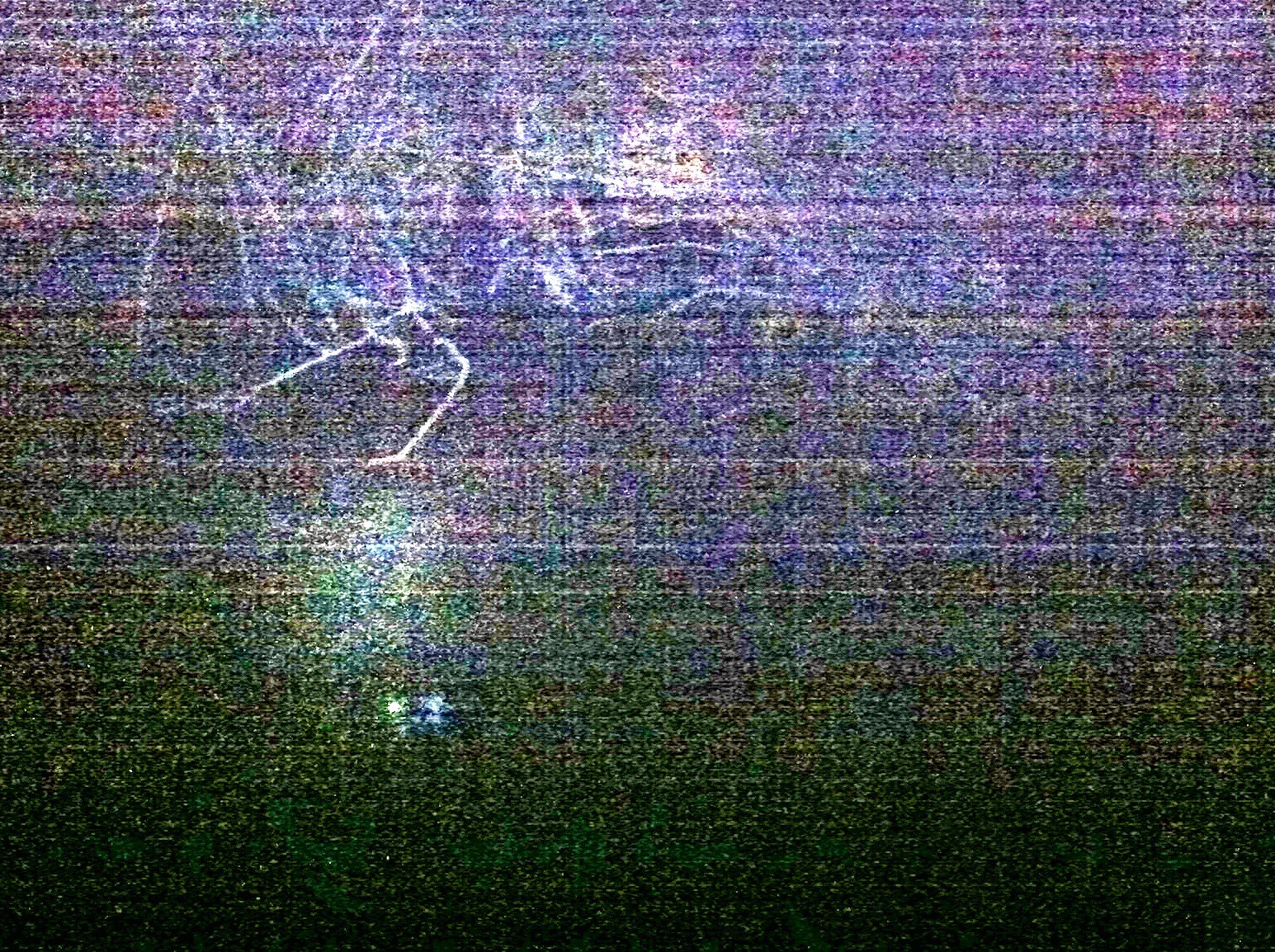The photograph depicts a heavily grainy and fuzzy image that combines elements suggesting both a distorted screen capture and a textured material. Horizontally, the image transitions from blue and purple hues at the top to greens, and finally to black at the bottom. This creates a gradient reminiscent of static on an old television with no signal. The image is chaotic, featuring horizontal lines and zigzag patterns, with white markings that could be interpreted as lightning or writing in the upper left corner, though they are obscured by the graininess.

Amidst the indistinct noise, the faint silhouette of a white skull appears in the upper middle section. Towards the lower part of the image on the left, there are two bright lights resembling car headlights, with another round, white light situated above them. The bottom section is especially complex, with suggestions of a faint tartan pattern in the fabric-like texture, showing colors transitioning from black to various shades of green. These details suggest possible wear and damage, perhaps from metallic objects abrading the material, adding to the overall disarray. The overall effect is a modern, abstract scene where distinct components are overlaid with pervasive static, creating a deeply fragmented visual experience.